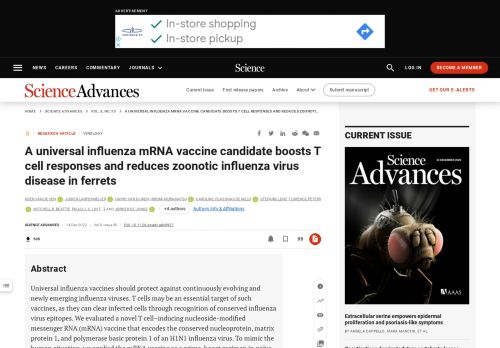This image is a screenshot from the Science Advances website. The top section of the webpage features a black header that includes various navigational elements. Centrally positioned within the header is a white rectangular advertisement adorned with a blue diamond icon, featuring a white circular arrow. 

Just below this advertisement, the site prominently displays the "Science Advances" title. The navigation bar beneath the title contains clickable sections labeled "Carrier," "Community," and "Journals," some of which have dropdown menus. To the far right is a conspicuous red button labeled "Become a Member," inviting visitors to join. An adjacent red text prompt reads "Get our e-alerts," offering subscription updates.

As you scroll down, the main content area features an article titled "A universal influenza mRNA vaccine candidate boosts T cell responses and reduces zoonotic influenza virus diseases in ferrets." Beneath the title, readers can access the abstract for a detailed overview of the research. To the right side of the page, the cover of the current issue is displayed, showcasing the striking image of an unusual-looking insect.